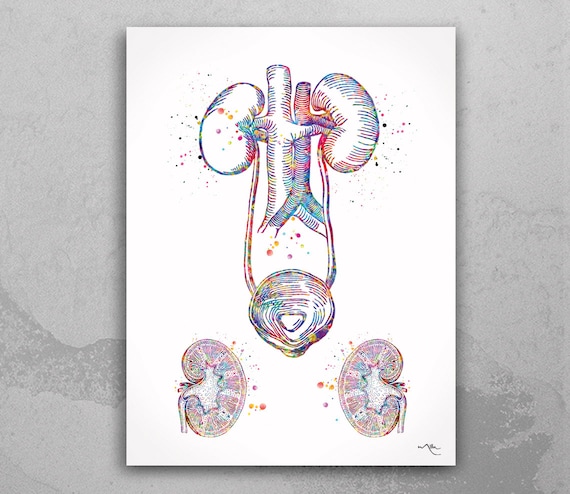This image is a vibrant and artistically stylized anatomical drawing, depicted on a white background laid over a gray, marble-like surface. The subject of the illustration appears to be a detailed study of human kidneys, despite some uncertainty among the describers. The drawing features two central organs, presumed to be kidneys, with tubes extending downward, suggesting a connection to the bladder. Additionally, there are cutaway sections showing the interior structures of the kidneys, positioned at the bottom of the image.

The artwork is strikingly colorful, employing a broad spectrum of rainbow hues. This use of color is reminiscent of a pen and ink technique but executed with exceptionally bright and varied tones. Reds, blues, purples, and other colors blend to create an eye-catching display. The names scribbled at the bottom of the drawing are illegible due to their small size. Notably, the drawing includes small dots or bubbles emanating from the illustrated organs, adding to the intricate detail of the piece. This artistic representation bridges medical illustration with a unique, colorful interpretation, making it as educational as it is visually captivating.